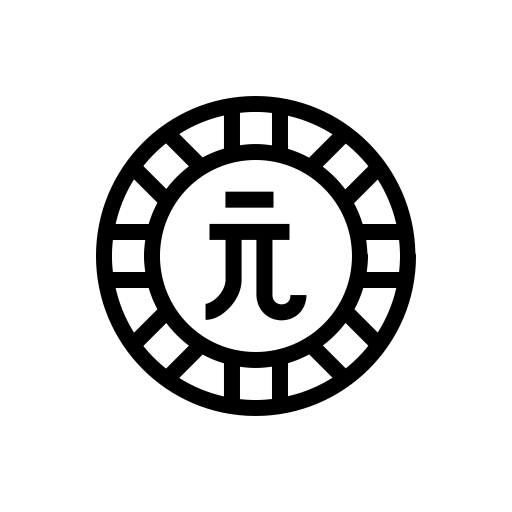The image depicts a logo consisting of two concentric circles on a white background. The outer circle has a dark black border, while the inner circle, also bordered in black, is notably smaller. Between these circles, there are about 14 to 16 black lines radiating outwards like spokes, giving the appearance of a wagon wheel. At the center of the inner circle, there is a symbol that resembles the mathematical symbol for pi (π) with a horizontal line or hyphen above it. Additionally, within the smaller circle, there's a J-shaped figure combined with a reversed J, together forming a shape akin to a fish hook. This intricate design could possibly be an old symbol with historical or cultural significance.